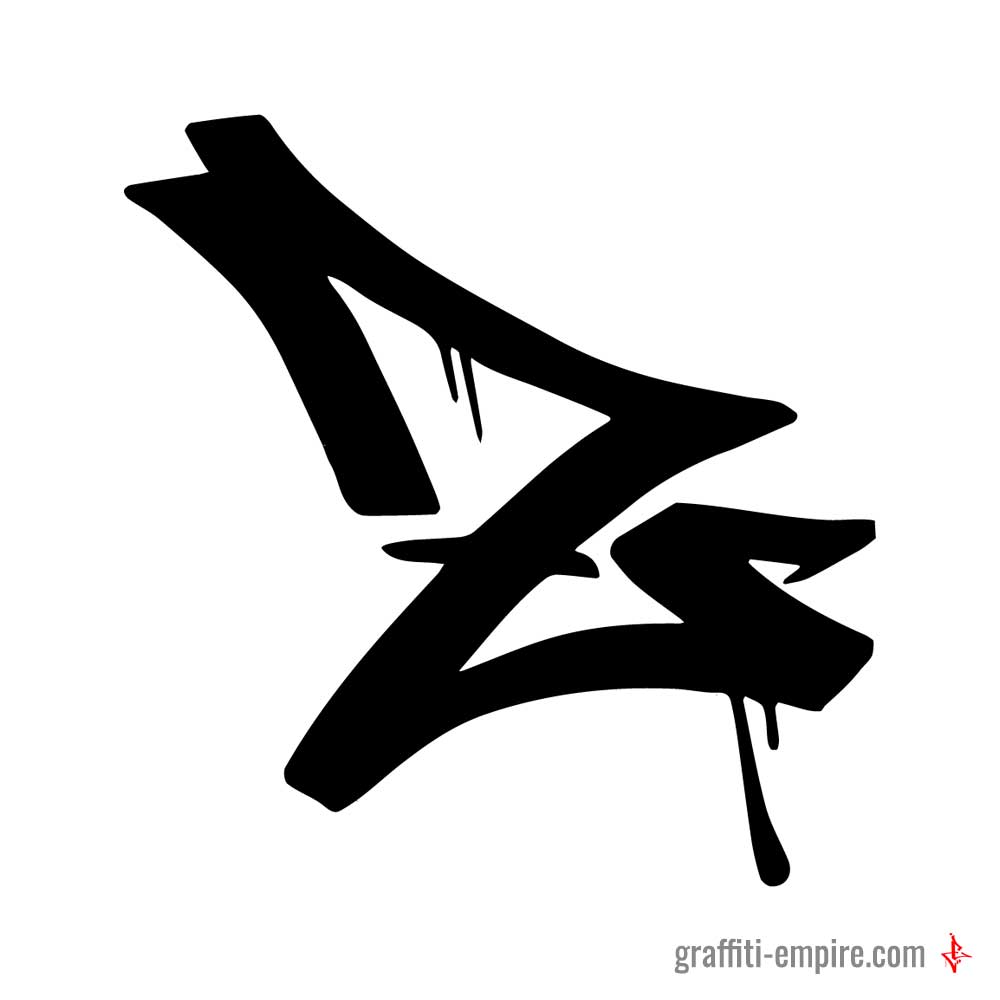The image features a bold, abstract design in black spray paint, prominently showcasing a distorted, jagged letter "Z" in a graffiti writing style. Dribbles of paint accentuate the piece, streaming down in various places on the Z. The design is monochrome, strictly black, contrasting sharply with the stark white background. It incorporates thorn-like protrusions on both sides of the Z, adding to its edgy, chaotic appearance. At the bottom of the image, "graffiti-empire.com" is referenced, accompanied by a similar symbol in red, resembling a fusion of a Z and a number seven. The overall effect is that of an intense, raw graffiti art piece, capturing the gritty essence of street art.